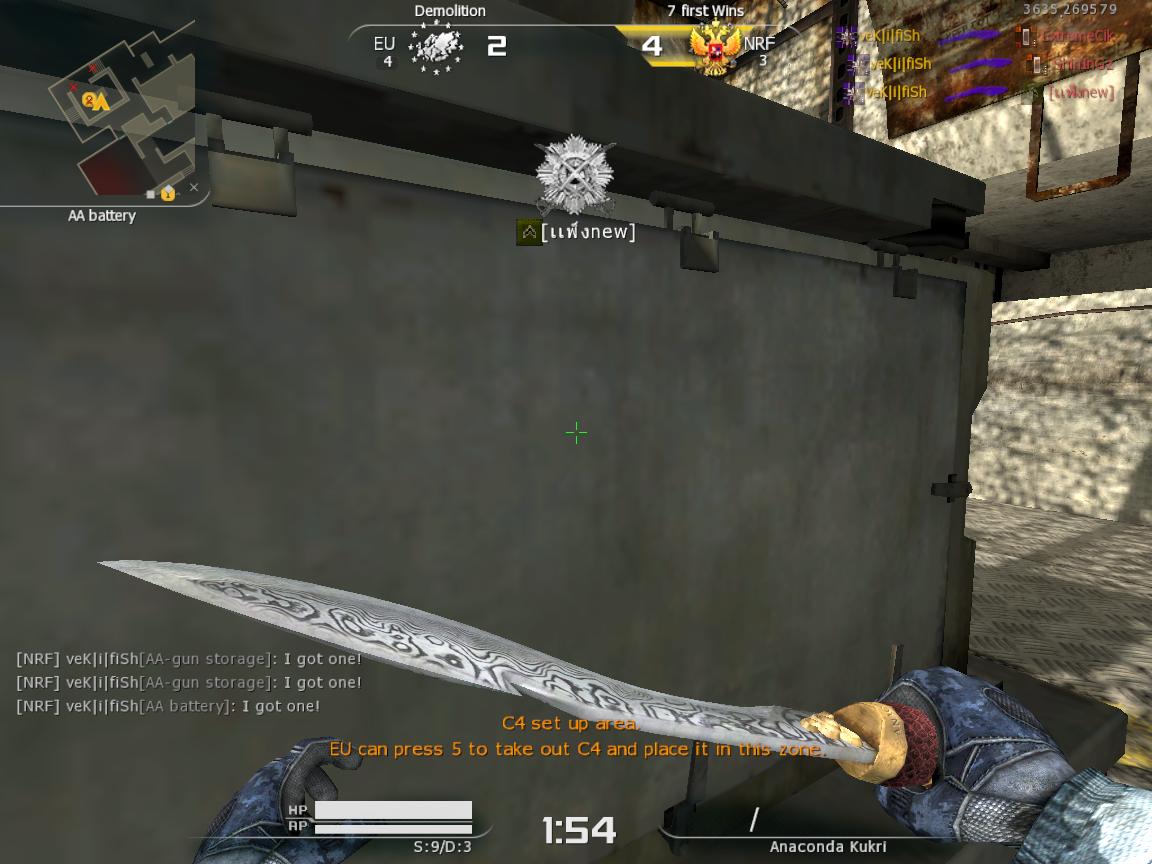This is an intricately detailed screenshot from a first-person shooter video game. The interface showcases several elements: in the upper left corner, there is a mini-map labeled "AA Battery" in white lettering. The bottom left corner contains a conversation log with repeating messages, such as "NRF VEK FISH AA GUN STORAGE. I got one!" and "NRF VEK FISH AA BATTERY I got one!" The central part of the screen highlights in orange text, "C4 SETUP AREA," indicating that players can press 5 to place C4 in this designated zone. A timer reading "1:54" is visible at the bottom center, likely a countdown. 

The main focus is a first-person view of the player's character, who is holding a combat knife named "Anaconda Kukri." The knife features a curved silver blade with ornate etchings, a golden hilt, and a red wrap. The character's hands are clad in blue camouflage gloves with green sleeves, and they seem to be standing in front of a gray object, possibly a wall, adorned with padlocks and a metal beam above it. Additional indicators show full HP and RP bars. The player's name is displayed in a foreign script, adding to the immersive experience.